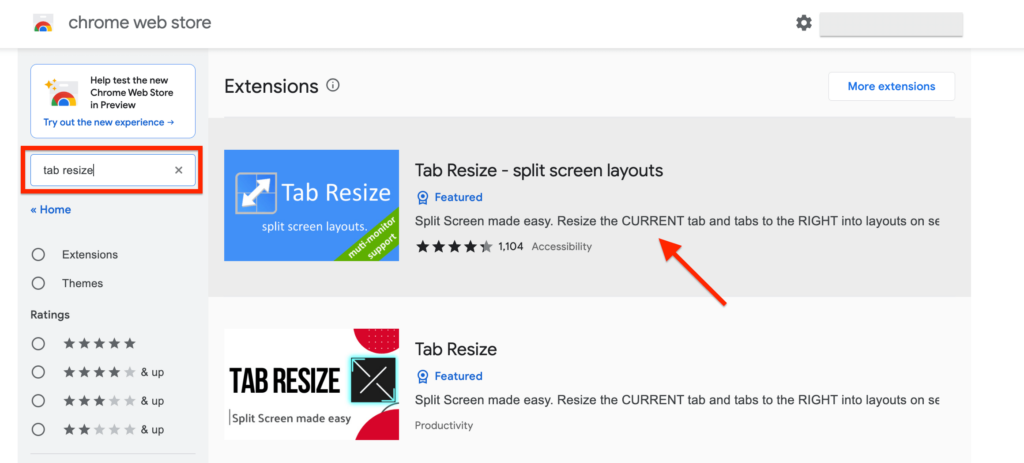In this detailed image of the Chrome Web Store interface, the header prominently displays the "Chrome Web Store" text in the top left corner alongside the Chrome Web Store logo. Adjacent to this, in the top right corner, there is a small search bar section, characterized by its grayish hue, accompanied by a gear icon to its left.

Directly below the main header, there is a highlighted box stating, "Help test the new Chrome Web Store in preview," with yet another Chrome Web Store logo to its left. Beneath this notification, a secondary search tab containing the term “Tab Resize” is visible, featuring an 'X' icon on its far right for clearing the search.

Moving further down, the interface is segmented into categories and filters. To the left, under the search area, are the labels “Extensions” and “Themes” with corresponding selection bubbles beside them. Below this category section, there is a "Ratings" filter with four selectable bubbles for five-star, four-star, three-star, and two-star ratings.

On the right side of the image, the word "Extensions" marks the section where two featured browser extensions are displayed. The first extension is titled "Tab Resize - Split Screen Layouts" and is labeled as "Featured" with a blue badge icon. Below it, the second extension simply named "Tab Resize" is listed without additional highlights.